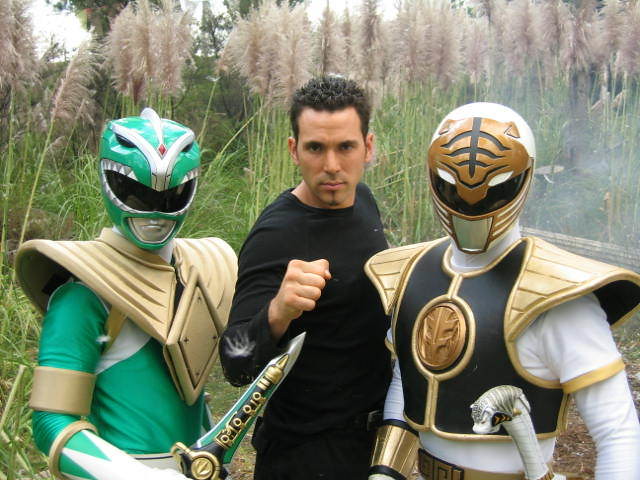In this square photograph, three individuals are positioned closely together in front of a backdrop of tall green blades of grass topped with brown feathery tips, with a bright white sky visible in the upper left and middle sections. The man in the center, dressed in a long-sleeved black shirt, has short spiky black hair and a serious expression. He is posing with his right fist raised towards the camera in a tough stance. On our left, the person to his right is dressed in a green Power Rangers uniform, featuring a green helmet with a black eye area outlined in silver, and gold armor over the chest and shoulders. This individual, possibly a woman, holds a black, green, and gold sword in their right hand, which is positioned near the man’s raised fist. To the man's left, on our right, stands another person in a white long-sleeved suit adorned with black and gold armor on the chest and shoulders, and a gold helmet. This figure holds a white rod topped with a snake’s head.